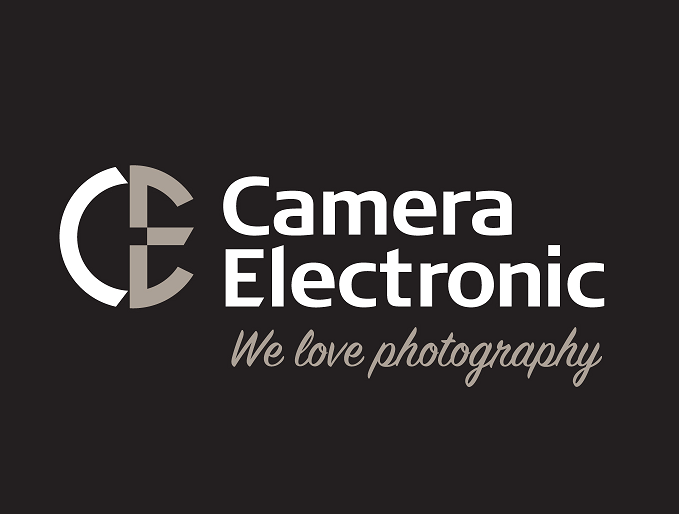The image features a company logo and text set against a completely black background. Positioned slightly left of center, the logo comprises stylized white 'C' and light grey 'E' letters. To the right of the logo, the text "Camera Electronics" is inscribed in white, and directly beneath it in light grey cursive are the words "We Love Photography." The layout suggests a professional design, likely intended for a business card or website, with a sophisticated interplay of black, white, and grey tones enhancing the elegant simplicity of the logo and text.